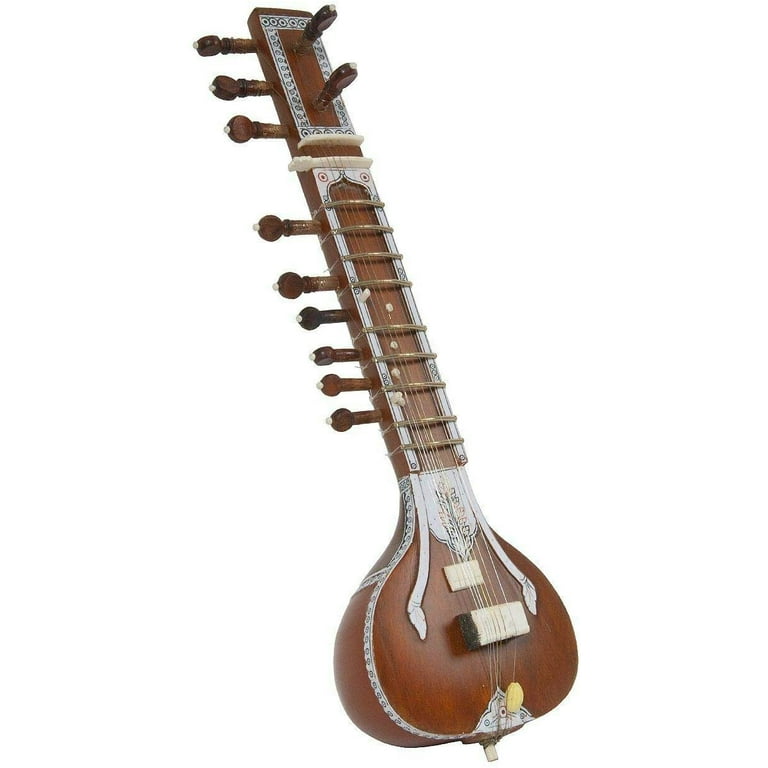This photograph showcases a sitar, a distinctly shaped musical instrument known for its long, wide neck and gourd-like base. The sitar features a deep mahogany color with elaborate silver embellishments along its edges. The silver detailing includes intricate floral patterns etched into the central metal parts and small circular designs that border the instrument. The sitar is adorned with multiple strings—seven or eight—each of which attaches to tuning knobs primarily located along the side of the neck, with two additional knobs facing outward at the top. The base of the instrument is adorned with a silver triangle and a brown oval-shaped object beneath the strings. Additional silver decorations continue up the neck, accentuating its length and elegance. There are also small dots on the neck, likely serving as markers or fretboard indicators. The image is focused solely on the sitar, presented against a plain background, emphasizing the intricate craftsmanship and ornate beauty of the instrument.